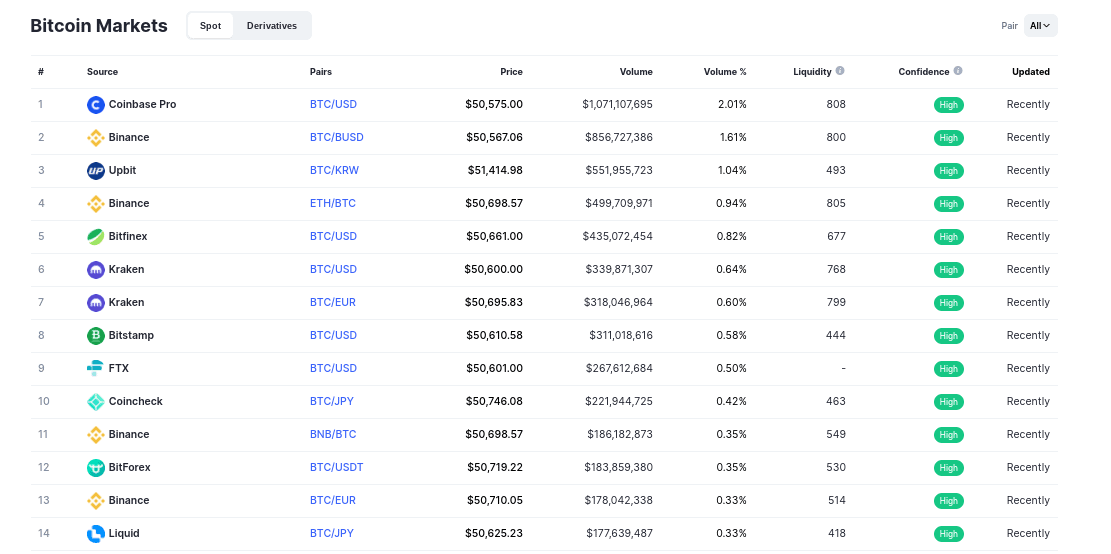The image depicts a web page displaying prices for various Bitcoin markets. It is wider than it is tall and has a white background that seamlessly merges into a more expansive layout. The page appears to be viewed on a computer rather than a mobile device. 

In the upper left-hand corner, the title "Bitcoin Markets" is prominently displayed, clearly indicating the focus of the page. To the right of the title, there are options to select between "Spot" and "Derivatives" markets, with the "Spot" market currently highlighted.

A detailed table occupies the majority of the page, with rows delineated by thin gray lines. The table includes several columns: Number, Source, Pairs, Price, Volume, Liquidity, Confidence, and Updated. Fourteen distinct Bitcoin markets are listed, featuring platforms such as Coinbase Pro, Binance, Upbit, Bitfinex, Kraken, Bitstamp, FTX, Coincheck, Bitforex, and Liquid, with Binance appearing multiple times.

For each market, the table provides the trading symbol, the current price of Bitcoin (hovering around $50,000), the total trading volume in dollars, the volume percentage, the liquidity score represented by a three-digit number, the confidence level (all marked as high), and the most recent update timestamp. Although specific dates are absent, the data reflects activity within the contemporary Bitcoin market landscape, likely within the past decade.